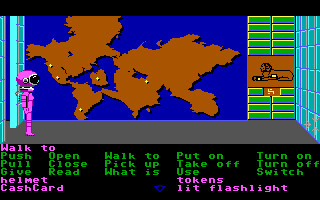The image is a detailed screenshot from a video game, framed by a thin black border at the top. The background prominently features a large blue area representing the ocean, overlaid with a flat, dark brown map of the world, speckled with a few yellow dots. To the right of this map, green rectangular bars display a central brown picture of an Egyptian sphinx facing left. Below the map and sphinx, there is a gray floor extending across the scene. On the left side of the map stands a pink astronaut, completely outfitted in a pink suit with a pink helmet and a black glass front, facing right. 

The bottom section of the image contains a black bar filled with various interactive text commands in pink and green. Commands include "Walk to," "Push," "Pull," "Give," "Open," "Close," "Read," "Pick Up," "What Is," "Put On," "Take Off," "Use," "Turn On," "Turn Off," and "Switch." Item options listed in pink include "Helmet," "Cash Card," "Tokens," and "Lit Flashlight," suggesting these items can be interacted with in the game's environment. The overall setup hints at a puzzle to be solved using these commands and items.